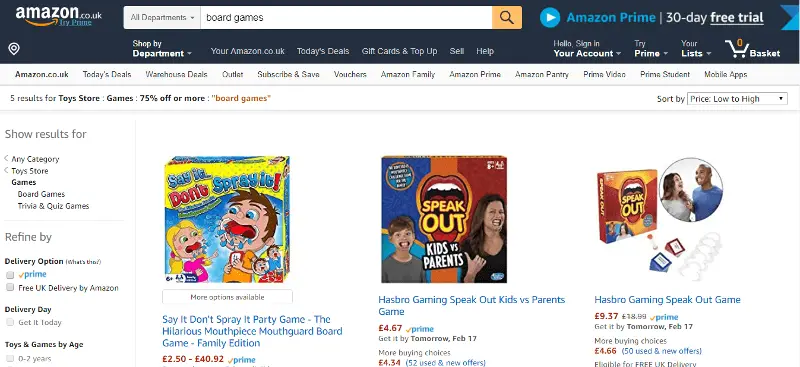This image displays the Amazon.co.uk website interface. In the top left corner, the recognizable Amazon name and logo are prominently featured against a dark blue backdrop. Centrally located in this panel is a white search bar, where users can input their search criteria. In this instance, a search for 'board games' across all departments has been executed.

Beneath the search bar, a results panel presents various headings along with the search outcomes. It notes that there are five listings in the Toy Store and Games category, showcasing discounts of up to 75%. Below these headings, three specific board games are prominently displayed with images and prices.

1. The first game, "Say It, Don't Spray It Party Game," is available at prices ranging from £2.50 to £40.92, suggesting a mix of new and second-hand options.
2. The second game, "Hasbro Gaming Speak Out Kids vs. Parents," is priced at £4.67 for Amazon Prime members, with additional new and used buying options starting at £4.34.
3. The final game, "Hasbro Gaming Speak Out," is listed at £9.37 for Prime members, with other new and used purchase options beginning at £4.66.

Each game's title, image, and fluctuating price options indicate varying conditions and seller offers, providing shoppers with a range of choices.